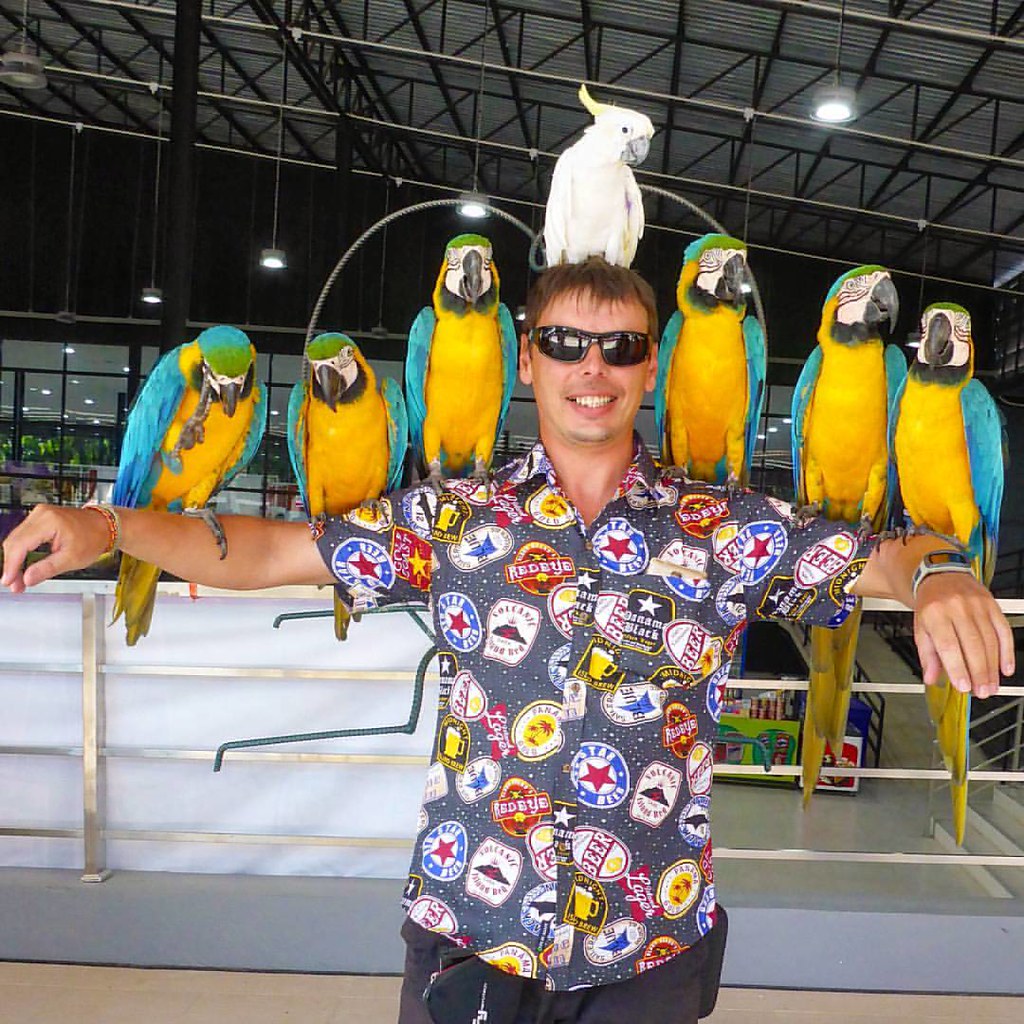In the photograph, a man stands with his arms spread out horizontally in a gymnasium or auditorium, under soft overhead lighting. He has short brown hair and is wearing blacked-out sunglasses, a busy patterned button-up shirt adorned with various beer bottle logos and colorful patches, as well as dark gray pants. His shirt breathes a vintage Hawaiian vibe, vibrant with red and blue logos.

Perched across his arms and head are seven striking parrots. Each arm balances three large parrots, their plumage a vivid combination of turquoise blue on the wings and crown, yellow on the body and sides of the head, and a green patch near the front. Their faces are marked with striking white areas around their black beaks. A stately white parrot rests atop his head, contrasting with the colorful array below. The man sports a watch on his left wrist and a big, joyous smile as he enjoys this vibrant display. Behind him, a silver railing is visible against a dark backdrop, with metal poles and ceiling lights faintly illuminating the scene.